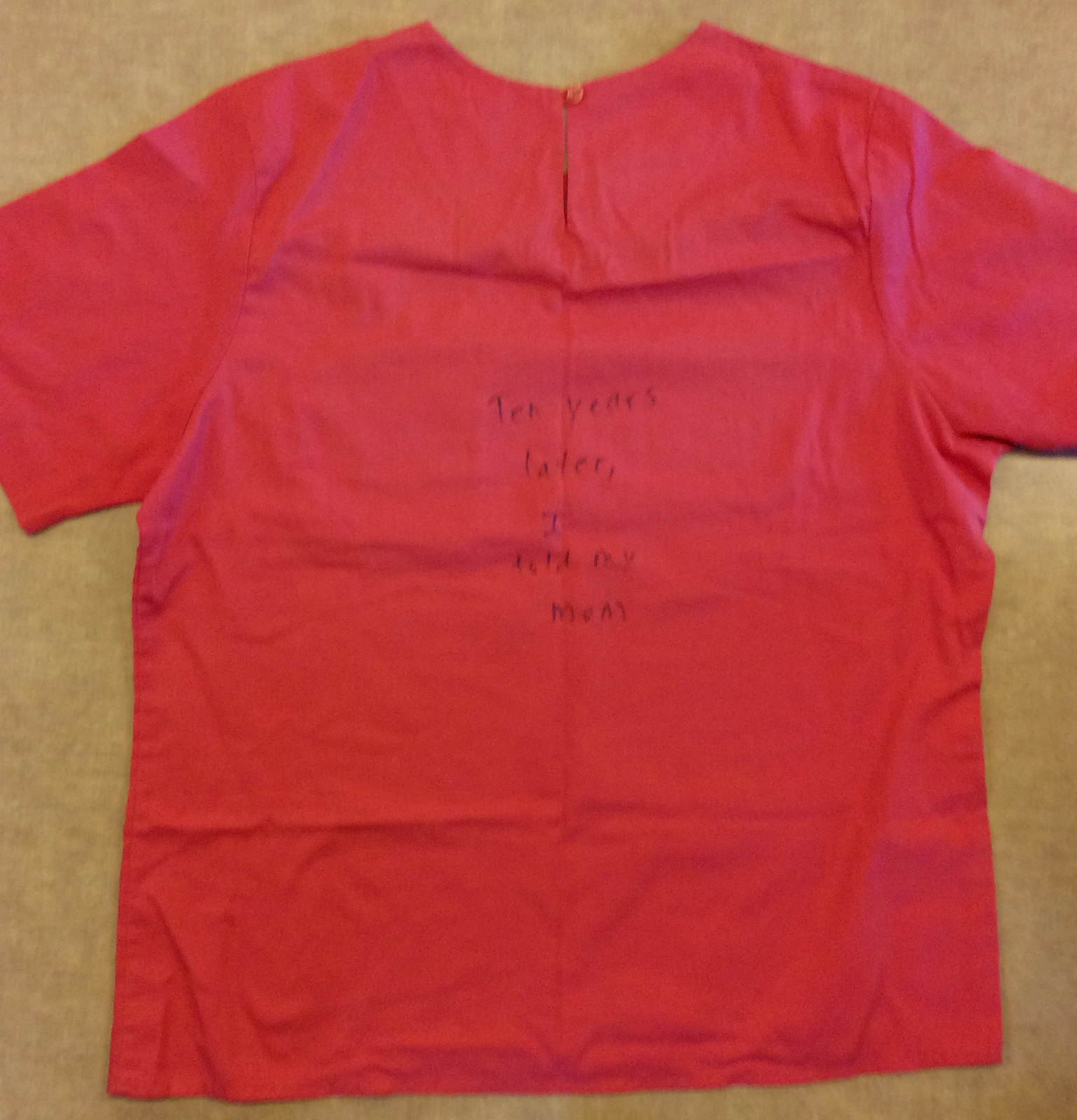This is a photograph of a coral-colored woman's short-sleeved shirt, displayed on a pale cream-colored surface, either a carpet or a table. The shirt features a single button at the collar, which secures the top of a slight slit below it. The fabric appears to have been folded multiple times before being laid out for the photo. There is handwritten text in ballpoint pen on the shirt that reads, "10 years later, I told my," with the last word being illegible.